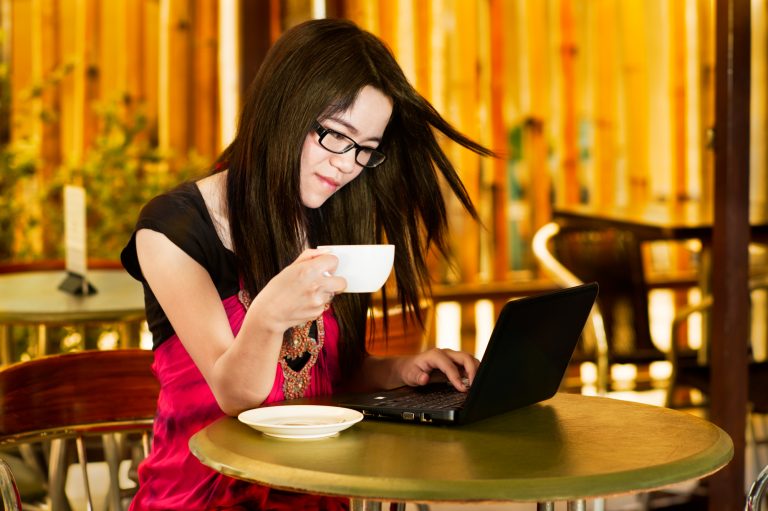In this image, a young Asian woman, possibly in her mid-20s, is seated at a small circular table with an olive green tabletop. She has long, straight black hair and wears black rectangular glasses. She is dressed in a short-sleeve top with fuchsia pink on the body and black straps over the shoulders. She is seated on a chair that has a red and off-yellow color scheme. The woman holds a white mug with her right hand, her elbow resting on the table, while typing on a black laptop with her left hand. A white saucer also sits on the table next to the laptop. In the background, there are several other tables and chairs, some wooden and others in plain brown wood. The background also features a wall that may be a dark orange color with visible beams extending from the ceiling, adding to the cozy ambiance of what appears to be a restaurant setting.